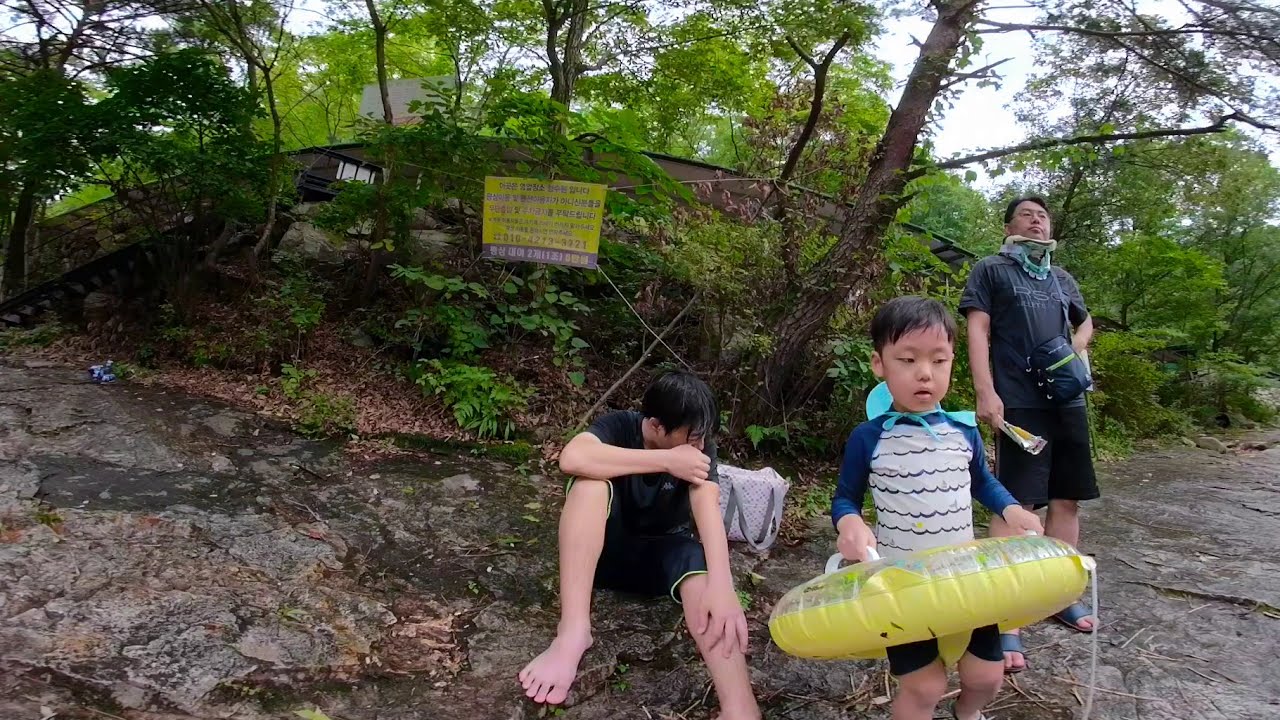In this image, set in a lush, wooded area with bright green foliage and several trees, three people are gathered on a rocky slope, likely near a river, as the two boys are wet and dressed in swim attire. To the rightmost part of the image stands an older Asian man, apparently in his fifties, carrying a blue bag around his neck and wearing a fanny pack. To his left is the smallest boy, a four or five-year-old, clad in a blue and white, long-sleeve swim shirt and black swim trunks. The child is standing within a yellow inner tube with two white handles, which he grasps. Sitting to the left is another boy, possibly a teenager, donning a dark shirt and black shorts. All of them appear to be tourists, with a backdrop featuring an arched brown bridge intertwined with vegetation. Behind them, tied to several trees, hangs a yellowish-green sign with a muted purple bottom, inscribed with what seems to be Chinese text, though it's blurry.